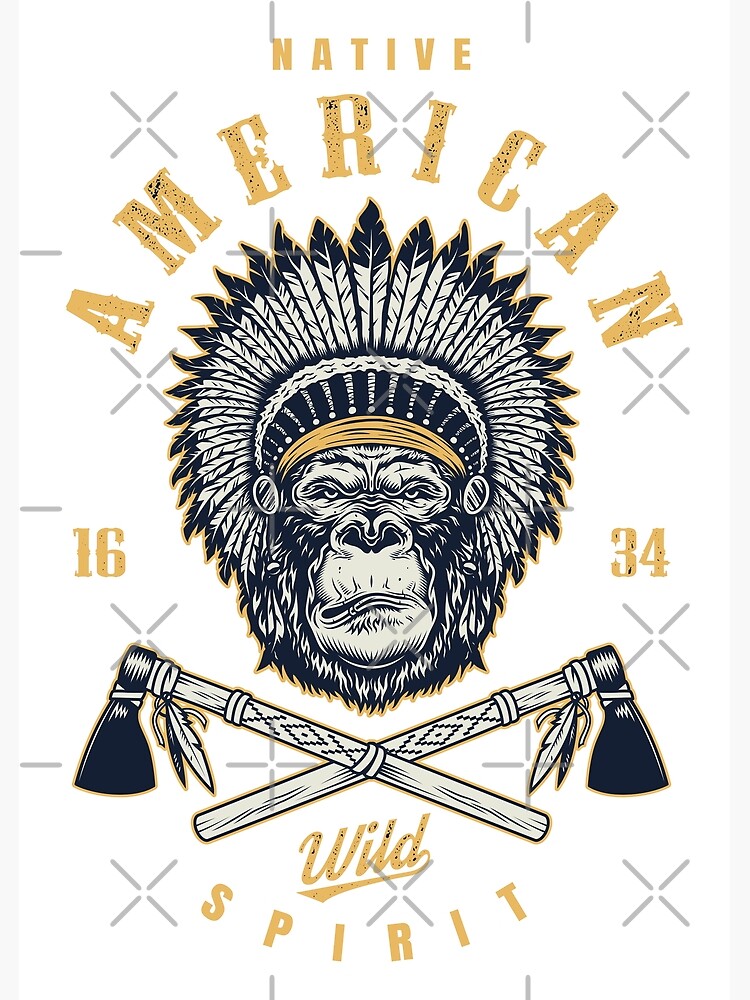This poster features a prominent Native American theme with an intricate design set against a white background. At the top, it reads "Native" in small yellow letters, followed by "American" in larger yellow letters arched above the center illustration. Dominating the central space is a detailed drawing of a chimpanzee wearing a traditional Native American headdress adorned with feathers. The feathers and the strip across the forehead feature touches of yellow or gold. Below the chimpanzee, two hatchets are crossed to form an X, each hatchet decorated with hanging feathers evocative of Native American artifacts. The left side of the image shows the number "16" while the right side shows "34". At the bottom, curving upward, it reads "Wild Spirit" in script, flanked by additional watermark-like images, including geometric shapes like X's and plus signs, which further enhance the cultural aesthetic.